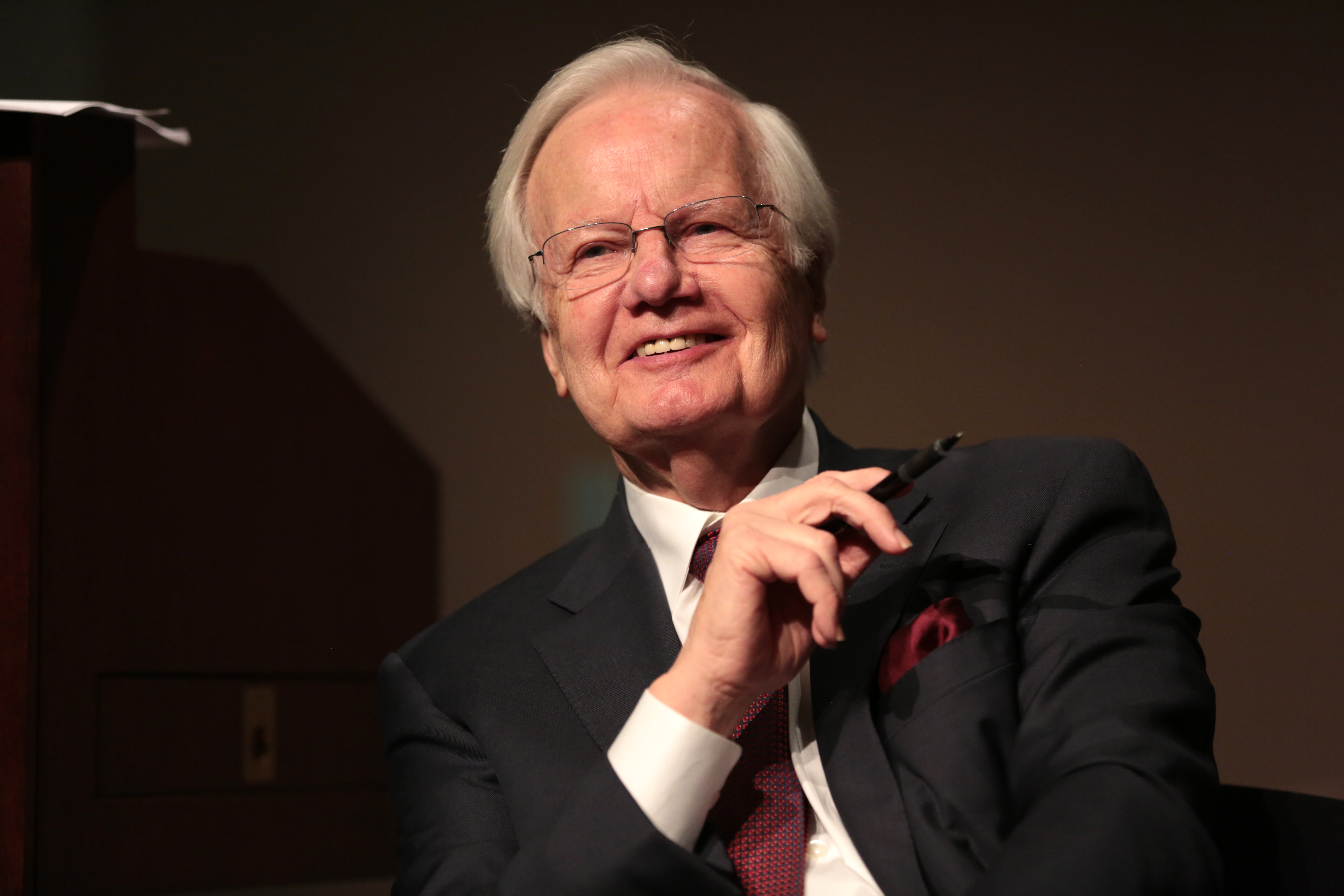In the image, an older gentleman of European descent is prominently featured against a dark background. He is seated in a chair, facing the camera, with a slight smile suggesting he is engaged in conversation or listening intently. His gray hair, short above the ears and parted to the side, frames his face. He wears thin wire-framed glasses which complement his distinguished appearance. 

He is dressed in a black suit with a white button-down shirt and a red tie adorned with small dots. A red handkerchief peaks out from his left chest pocket, adding a touch of color to his attire. In his right hand, held between his index and middle fingers, is a black cartridge pen, poised as if ready to write. His left arm rests by his side. A piece of paper on a stand or podium is faintly visible in the background, possibly indicating a professional setting. The scene is well-composed, capturing both the gentleman's poised demeanor and the subtle details of his surroundings.